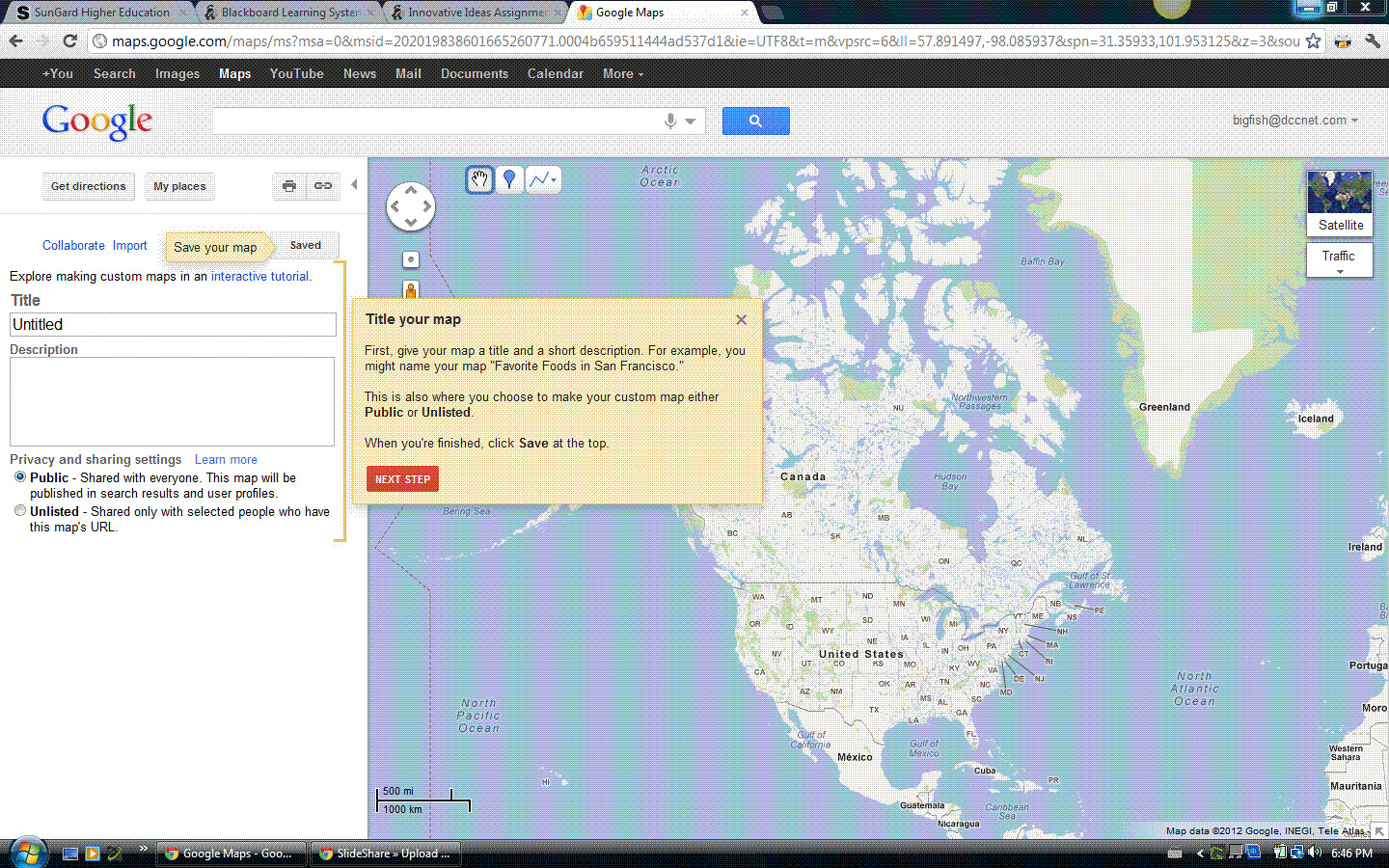The image is a pixelated computer screenshot of Google Maps on a screen. The interface displays various regions including the United States, Canada, Mexico, and Greenland. At the top, the Google logo is visible, indicating it is an older version of the site. Centered within the map interface, there is a prominent yellow box that contains instructions for titling the map and providing a short description, with an example suggesting "Favorite Foods in San Francisco." This yellow box also includes an option to make the custom map either public or unlisted, with a red box labeled "next step" and a double-sided yellow arrow pointing towards a white "saved" button. Additionally, the interface shows several options such as Get Directions, My Places, Collaborate, Import, Save Your Map, Saved, Explore, Making Custom Maps in an Interactive Tutorial, and privacy settings where the user has chosen to share the map publicly.